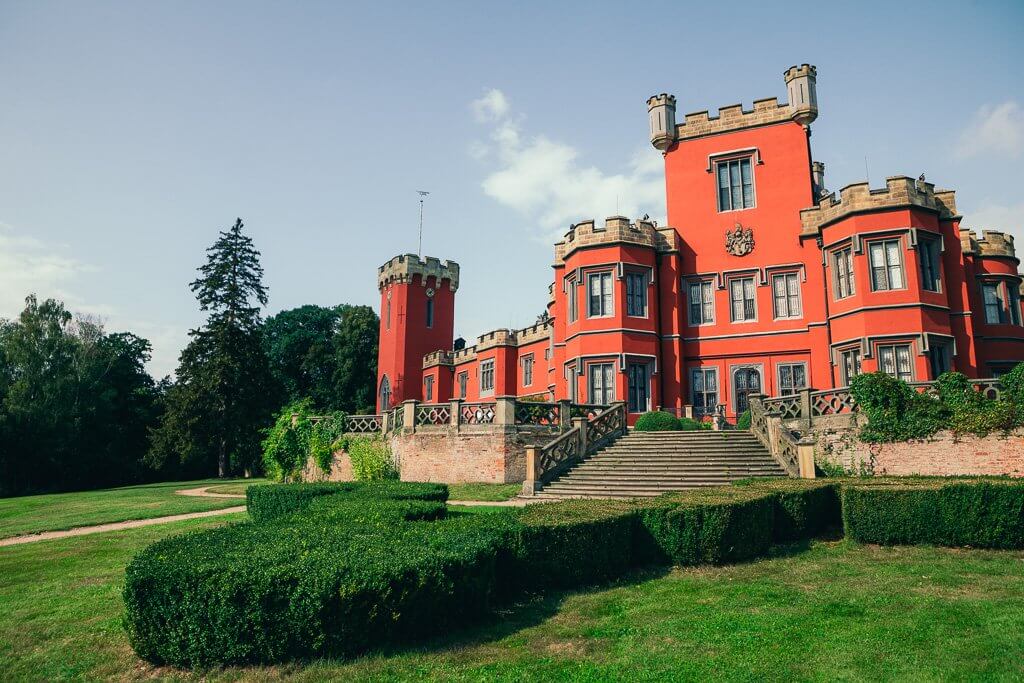The image showcases an elegant estate designed to resemble a historic castle, characterized by its distinct architectural features and vibrant color scheme. Set amidst a meticulously maintained green yard with perfectly trimmed, circular hedges, the estate is approached via a grand set of light brown, narrow stairs leading to a concrete patio with a decorative stone railing. The main building, bright red in color with beige trim that mimics castle brickwork, prominently features numerous large, four-pane, rectangular windows and boasts a unique combination of two and three-story sections, including an additional tower-like structure on the left side that houses a TV antenna. The entrance is marked by a curved front door, and there are intricate diamond-shaped patterns and vines adorning the brick walls. A badge resembling a horse is also discernible on the façade. In the background, lush green trees of varying sizes frame the scene against a bright blue sky dotted with a few white clouds. While the lawn appears vast and consists mostly of vibrant green grass, some brown patches are noticeable, adding a touch of natural imperfection to the picturesque setting.